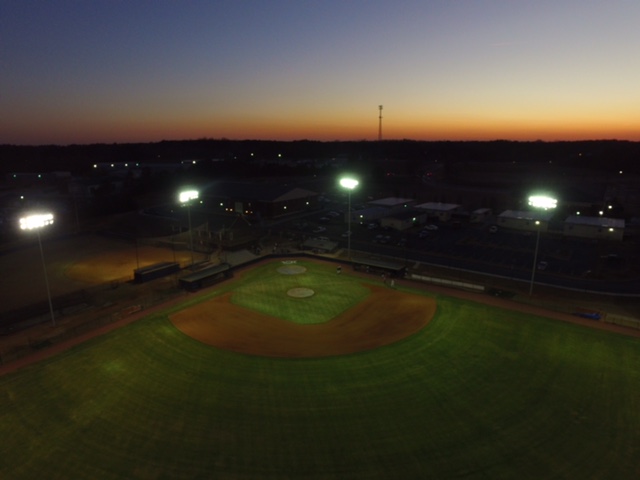This nighttime photograph captures a serene baseball stadium, bathed in the soft, ambient glow of a dusky sky. The horizon is painted in stunning gradients—from deep blue to white, yellow, and orange—marking the sun's recent descent. The field itself is meticulously maintained, showcasing the vibrant green outfield and the distinct brown dirt of the infield, with a whiter pitching mound. Four towering floodlights cast their beams brilliantly, highlighting the diamond shape of the field and sections of the outfield. Surrounding the field is a boundary fence, beyond which lies the cityscape, dotted with illuminated buildings and sporadic lights. The skyline features an assortment of structures, including a prominent tall tower and several white buildings, while a large, darker building stands directly behind home plate. The scene also includes glimpses of a parking lot and distant cars, testament to the quiet yet alive urban environment surrounding this peaceful baseball sanctuary.